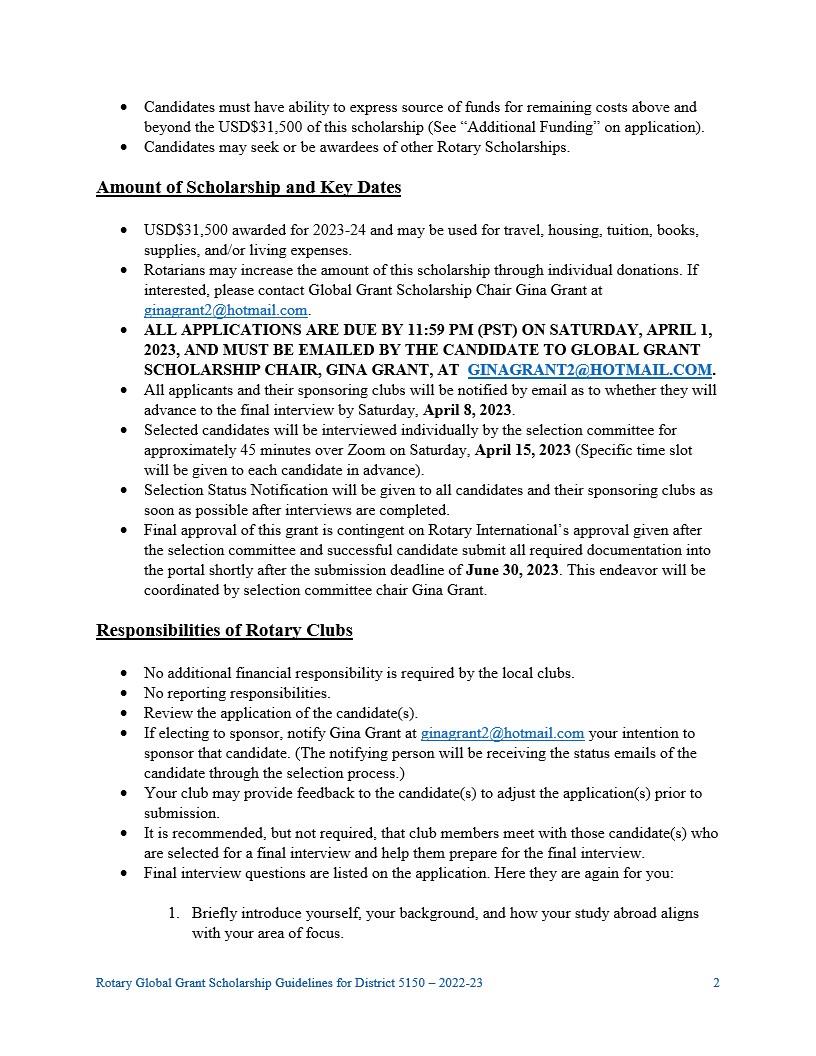**Detailed Caption:**

The image is a screenshot of a document which does not include the document title. 

- The first section contains bullet points:
  - The first bullet point states that "Candidates must have the ability to express the source of funds for remaining costs above and beyond $31,500 of the scholarship (see additional funding on application)."
  - The second bullet point mentions that "Candidates may seek to or be awardees of other Rotary scholarships."

- The next section titled "Amount of Scholarship and Key Dates" is underlined and contains eight bullet points.
  - Within this section, there is an underlined email hyperlink: GinaGrant2@hotmail.com.
  - The word "Candidates" appears again within the second and third bullet points.

- The following section, "Responsibilities of Rotary Clubs," is both bolded and underlined. 
  - This section lists around seven bullet points.
  - The email address GinaGrant2@hotmail.com appears again in the fourth bullet point.

At the bottom left of the document, in very small white text, it says, "Rotary Global Grant Scholarship Guidelines for District 5150, 2022 to 2023." In the far right corner, there is the number "2."